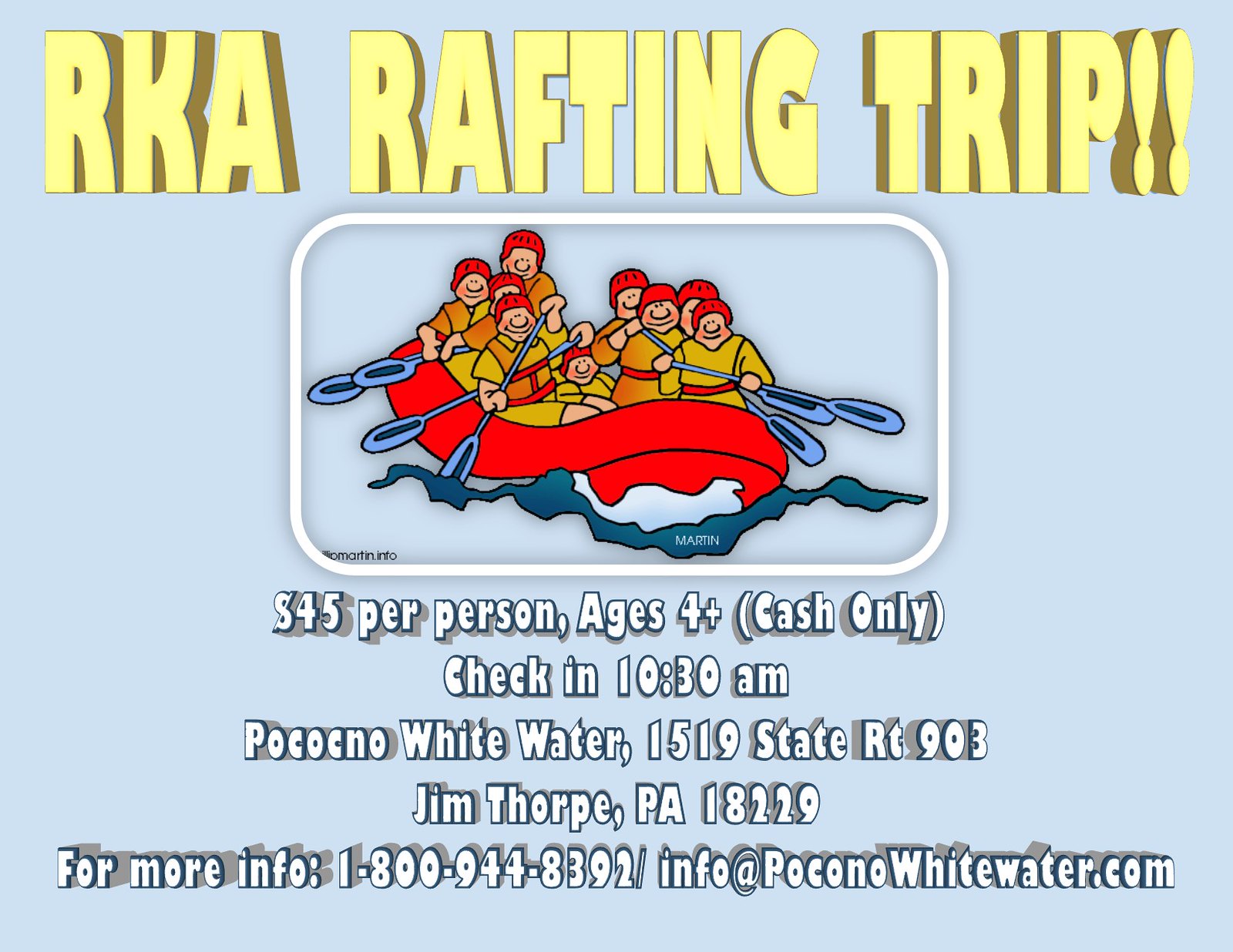The image is an advertisement for the "RKA Rafting Trip!" emblazoned at the top in gold, 3D text, accompanied by two exclamation points. Directly beneath the heading is a simple cartoon drawing of people rafting. They are navigating a river in a red raft, dressed in beige rafting suits with red helmets, holding blue paddles. The water is depicted in light blue, suggesting a lively excursion in a natural setting. Below the illustration, detailed trip information is provided in white text against a light blue backdrop. The trip costs $45 per person and is available for individuals aged 4 and up, with cash being the only accepted payment method. Check-in time is stated as 10:30 a.m. The location for the adventure is Pocono Whitewater, situated at 1519 State Route 903, Jim Thorpe, PA 18229. For additional information, a contact number, 1-800-944-8392, and an email address, info@PoconoWhitewater.com, are provided.